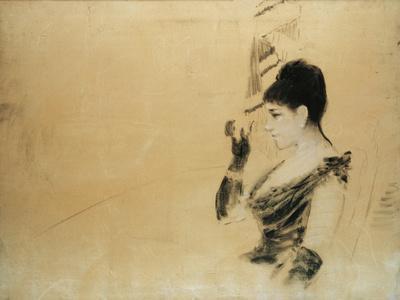The image is a wide, landscape-oriented drawing on an off-white, cream-colored background, with noticeable eraser marks and smudges. Dominating the right-hand side is a detailed, unfinished sketch of a Caucasian woman in profile. She has dark hair pulled up into a bun and is adorned with an earring. The woman wears an elegant, low-cut, short-sleeved, or potentially a boat neck dress or gown paired with long gloves that extend to her elbows. In the drawing, her left arm is positioned down, revealing some glove and possibly a bracelet or watch with a distinctive cream mark, while her right arm is bent, with her hand near her face. The sketch includes some background elements like a shaded area above her head, which could suggest a chair, furniture, or a window, though these elements remain ambiguous and slightly abstract. The image is devoid of other characters or text and seems to be an initial phase of a more intricate artwork.